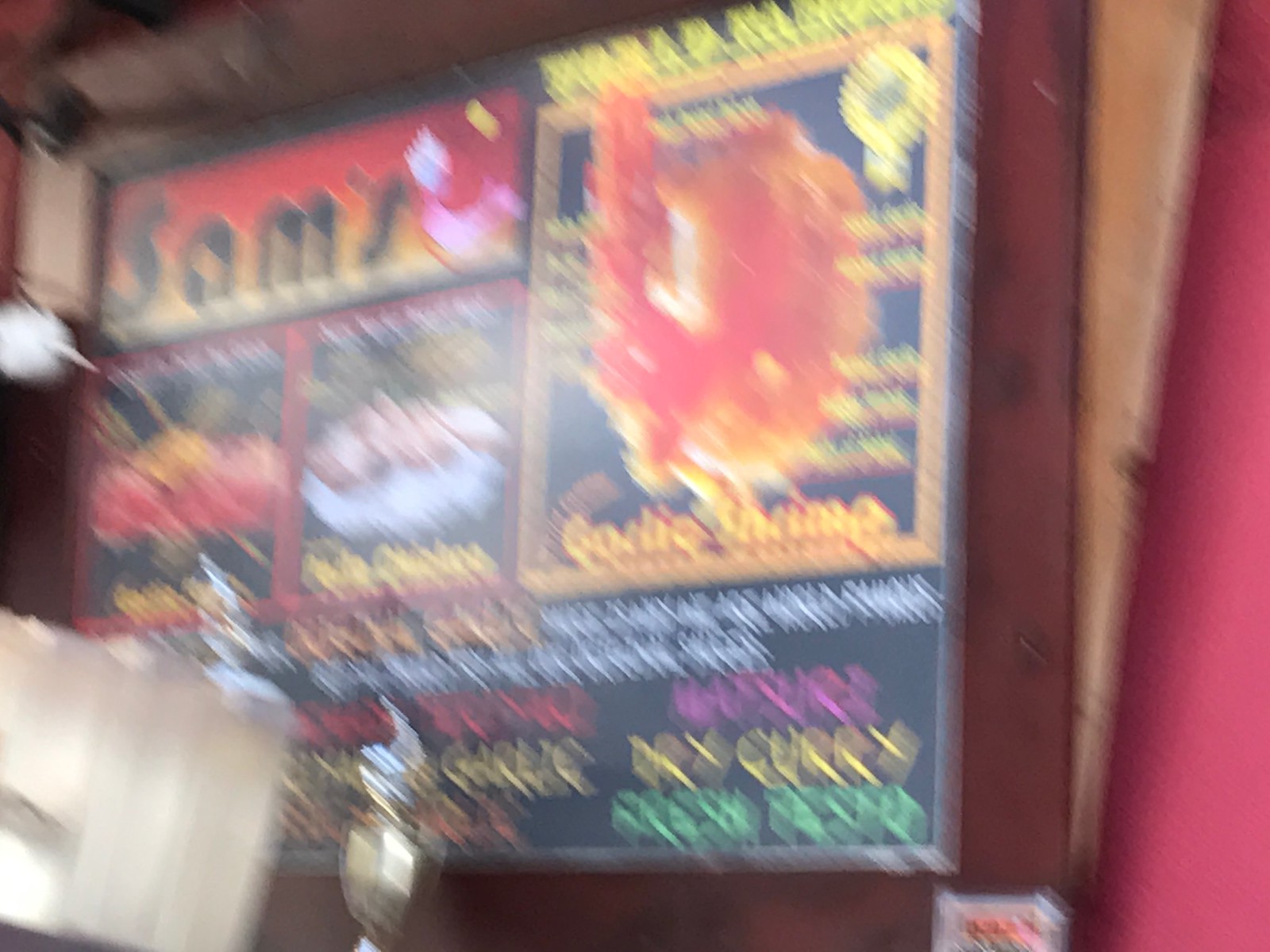The blurred image depicts a colorful restaurant menu board, prominently titled "Sam's" in the upper left corner. The sign exhibits a vivid array of reds, yellows, purples, greens, and oranges, hinting at an Indian or possibly Chinese cuisine with menu highlights such as "garlic shrimp curry" and the word "fresh." The board appears to have various sections, with notable yellow writing and possibly pictures of food, but the blur makes it challenging to distinguish specifics. The surrounding environment includes a red backdrop with beige elements, and the foreground features a white, cylindrically shaped object, potentially indicative of stacked buckets, a pipe, or an adjustable hose. The entire image is streaky due to motion blur, suggesting the photographer struggled with a steady hand or low shutter speed.